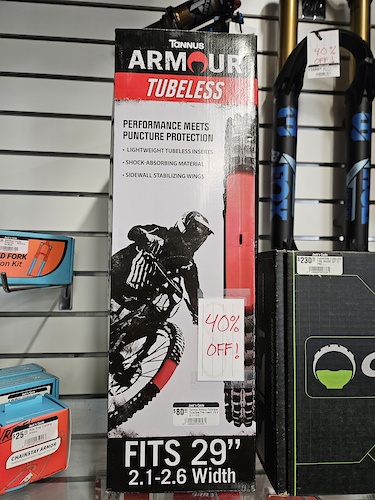The image captures a section of a store, likely a hardware or bike shop, focusing on a product display mounted on a white shiplap wall. Central to the image is a portrait-layout box prominently highlighted, primarily black and red in color, with white and gray text. The top part of the box displays the brand name "Tannis Arbor," followed by text that reads "tubeless" on a red background. Further down, it boasts "performance meets puncture protection," accompanied by three bullet points elaborating on its features. An illustration of a cyclist is depicted below the text. A white paper with red writing, taped onto the product, announces a "40% off" discount. The box also indicates its compatibility with 29-inch tires, ranging from 2.1 to 2.6 inches in width. Adjacent to this primary product, other items are visible but partly cut off. To the right is a black item with blue lettering, possibly a bike lock, and to the left are two smaller boxes in blue and corally peach hues. These details collectively suggest a well-organized retail space focused on cycling accessories.